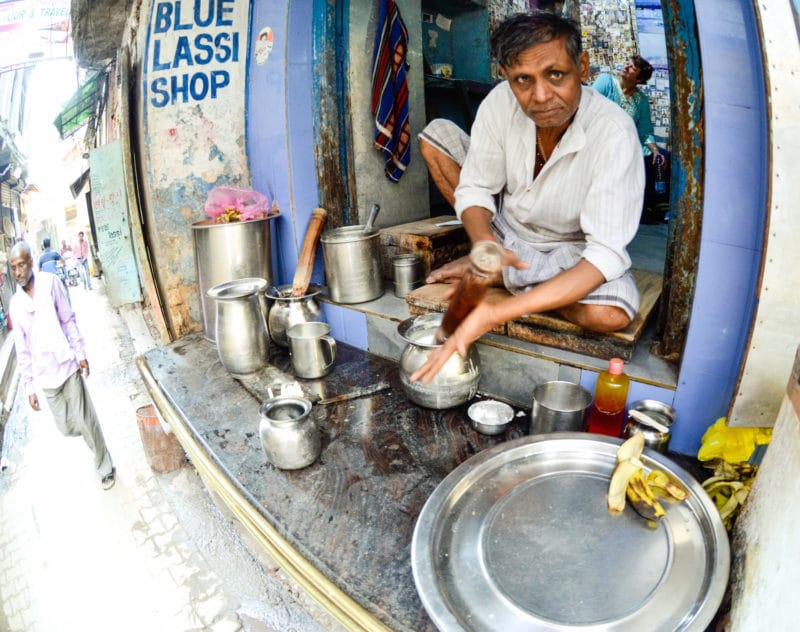In the photo, a middle-aged, dark-skinned man, possibly from India, is seated in his worn and weathered shop named "Blue Lassie Shop," as indicated by a distressed blue sign on the side. The man, dressed in a long, white robe-like shirt, is sitting cross-legged on a floor cushion. His hair is messy, and he is fully engaged in his task, looking directly at the camera with a glass container holding a dark brown liquid in one hand. Surrounding him on various levels are several large silver containers and bowls, along with a round tray that has a half-eaten banana on it. Beside him, there are several other bottles of liquid. The shop is located in a bustling, village-like shopping district, possibly an alley in a city like Delhi. The photo captures the busy ambience of the area, with a few other people visible in the background. The man appears to be preparing food, possibly crushing or mixing something in one of the steel bowls with a wooden object.